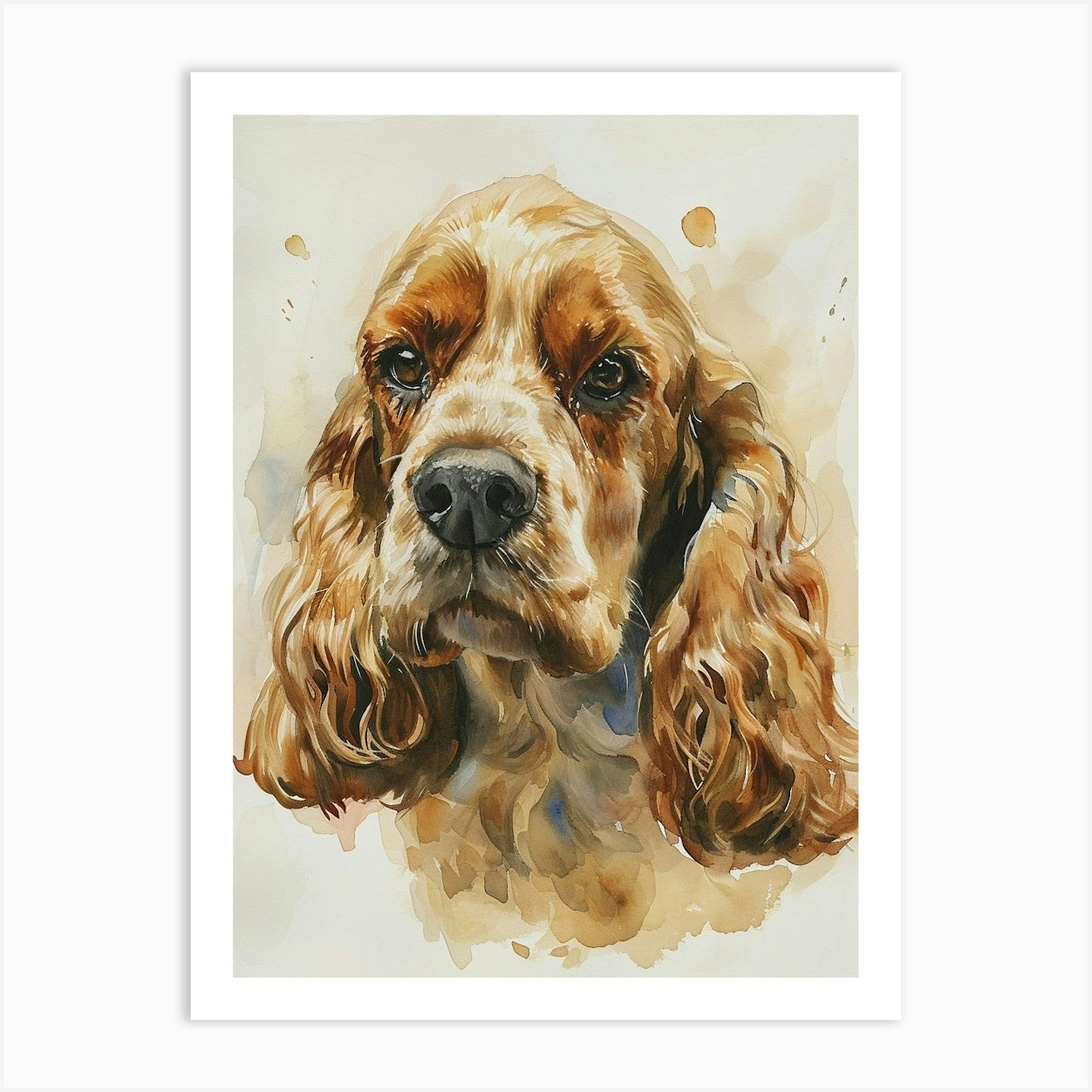This is a detailed watercolor painting of a Cocker Spaniel, framed by a white border. The artwork prominently features the dog's head, with its expressive brown eyes, black nose, and long, curly ears hanging well below its mouth. The dog’s face is predominantly a light brown to amber hue, with a mix of tan and small spots of darker brown on the muzzle and around the eyes. Below the chin, the chest area becomes more abstract with brush strokes in brown and hints of blue. The background is primarily a light brown, complemented by watercolor spots that add depth and texture. Above the dog's head, subtle paint splatters contribute to the artistic, messy style of the painting. The overall composition captures a relaxed and beautiful essence of the spaniel.